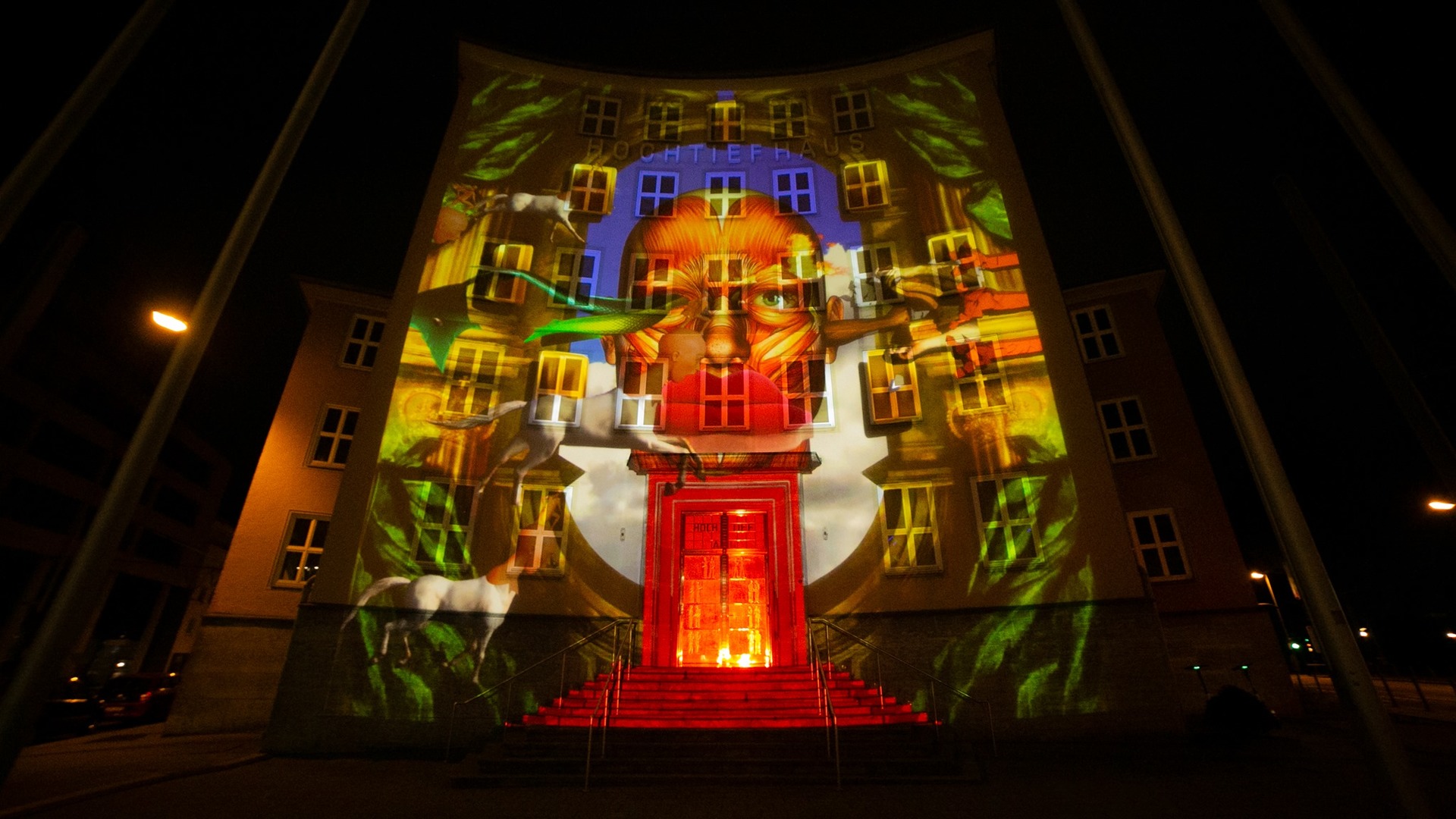The image depicts a tall building at night, adorned with a vivid projection of an elderly man's face. The man, likely Caucasian, has tanned skin and a white beard. The face, which appears to be orange-colored, is framed by a blue, rounded shape and extends over the building's windows. Below the face, a red structure that resembles a door adds to the striking visual. The background features a dark, black sky, with streetlights and parked vehicles visible. Additionally, the building's brown exterior and glass-pane windows are partially visible under the projection, contributing to the structure's unique aesthetic. Scattered greenery and hints of animals and birds add further detail to the scene.